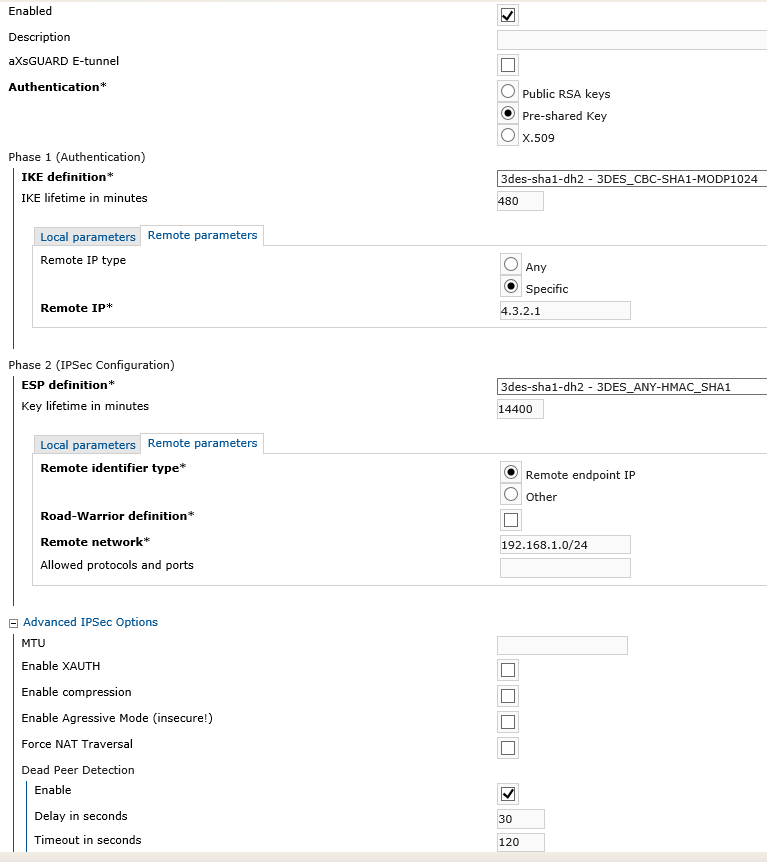This image presents detailed information about computer communication and security settings, specifically related to an AXSGUARD E-Tunnel configuration on a white background with predominantly black text and sections highlighted in blue.

At the top left corner, the word "Enabled" is displayed in black text. Below it, the section titled "Description" appears, followed by the alphanumeric string "AXSGUARD E-Tunnel." Underneath, the bold text "Authentication" is accompanied by an asterisk. Adjacent to this section on the right, there is a checkbox, an open gray box, and an unchecked white box. 

Below this, three white circles with gray rectangular backgrounds present different authentication methods. The top circle is labeled "Public RSA Keys," the middle circle "Pre-Shared Key" (which is checked and contains a small black circle in its center), and the bottom circle "X.509."

The second main section begins with "Phase 1 Authentication," followed by "IKE Definition" and "IKE Lifetime in Minutes." This section includes rectangular segments for "Local Parameters" and "Remote Parameters," the latter being highlighted in white.

Within the "Remote Parameters" subsection, there are items like "Remote IP Type" and "Remote IP," coupled with a checkbox that offers options "Any" or "Specific," followed by the IP address "4.3.2.1."

The following section labeled "Phase 2 (IPSEC Configuration)" mirrors the structure of the preceding sections with similar textual elements. In the highlighted white "Remote Parameters" box, it lists items such as "Remote Identifier Type," "Road Warrior Definition," "Remote Network," and "Allow Protocols and Ports."

Towards the bottom, the section titled "Advanced IPSEC Options" is highlighted in blue, encompassing various settings. Items listed include "MTU," "Enable XAU-Auth," "Enable Compression," "Enable Aggressive Mode," "Force NAT Traversal," "Dead Peer Detection," "Enable Delay in Seconds," and "Timeout in Seconds." Each of these items has corresponding checkboxes to the right that are either checked or left open.